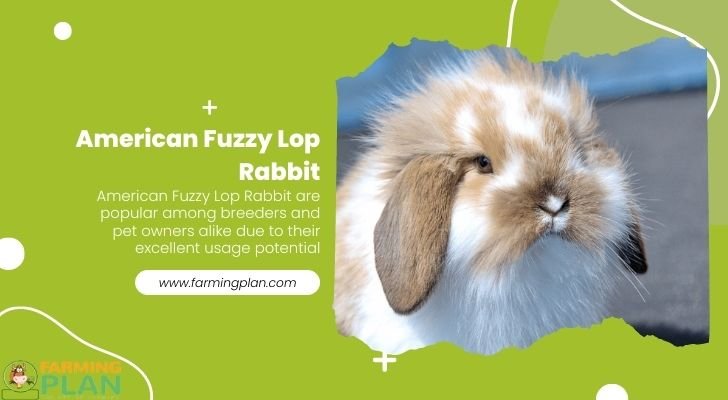The image displays a website homepage featuring a prominently placed, partially tattered photograph of an American Fuzzy Lop Rabbit. The photograph appears deliberately ripped at the top and bottom edges, while the sides remain crisp and straight. The rabbit showcased in the picture exhibits droopy ears, predominantly white fur with hints of light brown, and striking white whiskers contrasted against its brown eyes. Its face has a distinctive, flat appearance reminiscent of a pug, lacking a pronounced muzzle.

Above the photograph, a plus sign is visible, followed by the text "American Fuzzy Lop Rabbit" in white letters. Further information describes the breed as popular among breeders and pet owners due to their excellent potential for various uses. At the bottom left corner of the homepage, within a white box, the website URL www.farmingplan.com is provided. Adjacent to this is an icon featuring a cow with the site name "Farming Plan."